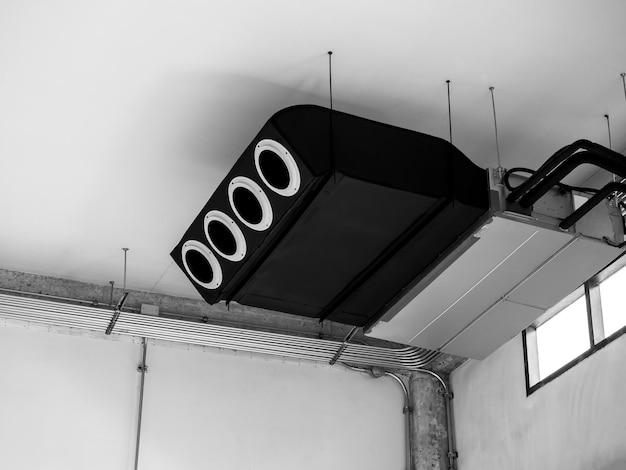The image is a detailed ceiling shot of a rectangular, black garage door opener mounted in an unfinished, possibly basement-like room. The opener features four round recess lights built into its underside and is securely attached to a white ceiling with small grey metal hangers. This industrial setting is further characterized by white or grey concrete walls and a network of grey or silver metal pipes running from the base of the machinery through the walls. These pipes are fastened to the ceiling with silver hangers, and additional pipes run down the wall in the corner. The room has two small, high-placed windows with black borders, which add a stark contrast to the otherwise monochromatic space. The overall shape of the image is wider than it is tall, highlighting the room’s width and the intricately mounted mechanical equipment.